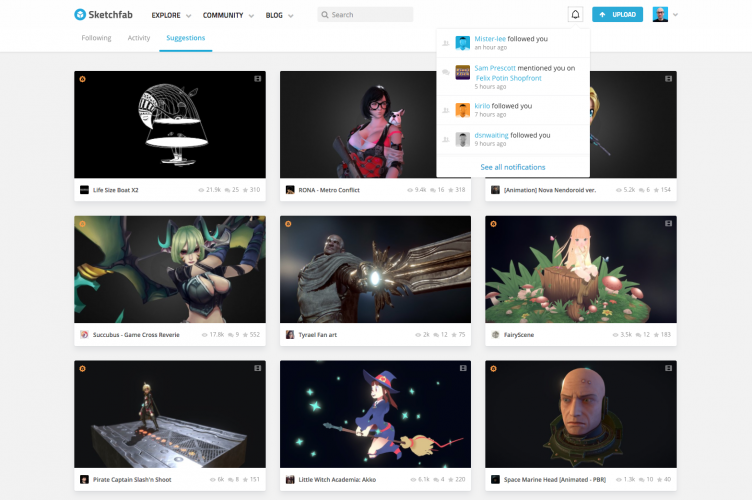The web page depicted is that of Sketchfab, an online platform for viewing and sharing 3D models. The upper section of the page features a sleek navigation bar set against a white background. The navigation bar includes the Sketchfab logo, followed by navigation options labeled "Explore," "Community," and "Blog," all rendered in uppercase black font. Adjacent to these options is a central search bar. Towards the right, there's a light blue "Upload" button with white text, and further to the right, a profile icon characterized by a man's head on a blue background.

The main content area of the screen displays a 3x3 grid of images, each set against a dark or black background. These images showcase a variety of subjects. The second image in the top row features a woman with black hair and glasses, clad in a low-cut black dress adorned with a red pattern on the front. She appears to possibly have a bird on her right shoulder, although it’s difficult to discern clearly. In the middle row, the first image on the left presents a woman with a blonde bob haircut, wearing a revealing top that accentuates her cleavage. The image extends down to show her midsection. The center image in the middle row depicts a large bald man positioned on the left side of the frame, brandishing an enormous sword with a reflective jaw at its base.